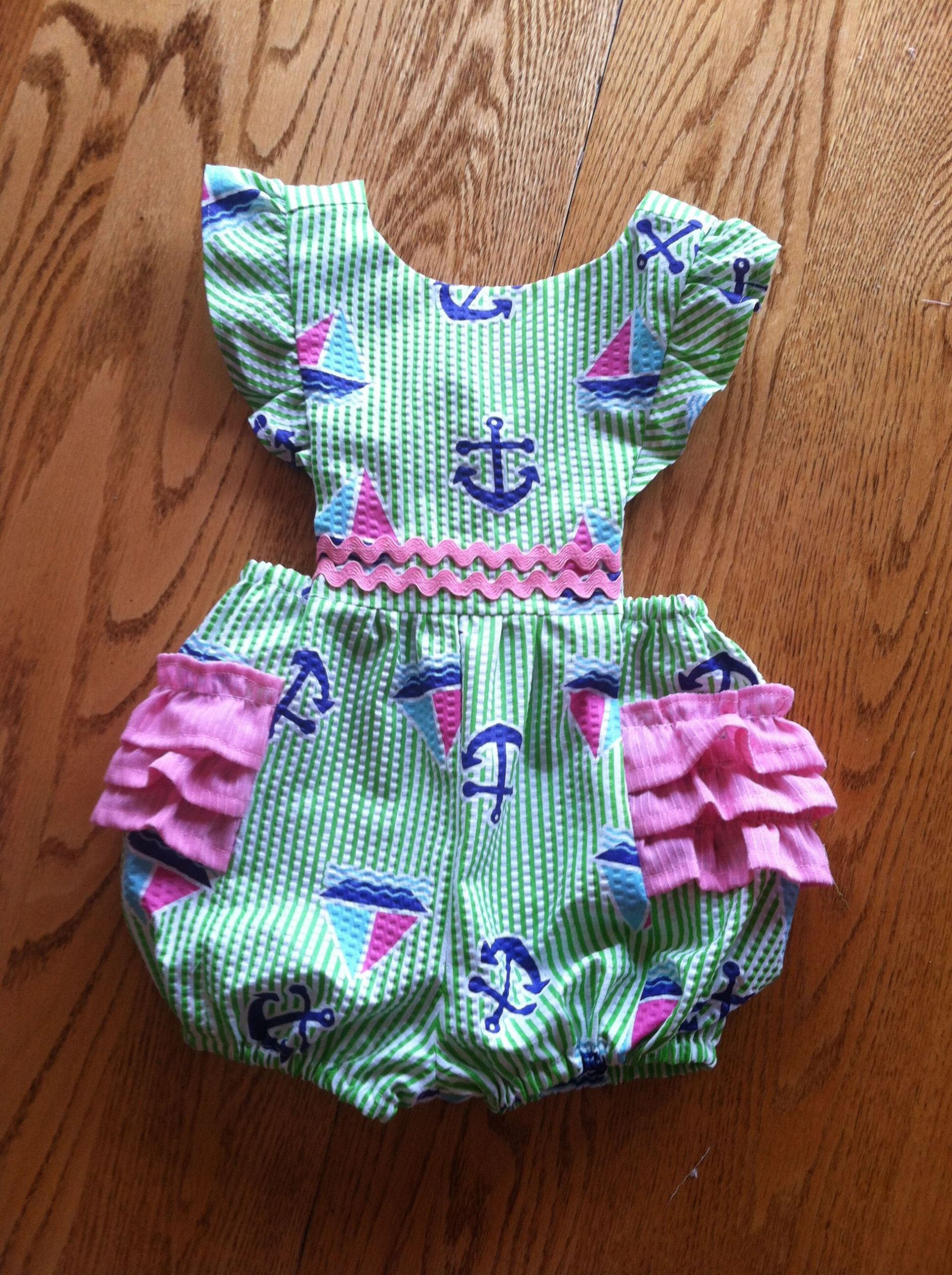In this indoor photograph, an infant girl's outfit, resembling a dress but functioning as a bathing suit, is displayed on a wooden surface with visible, textured grains in various shades of brown. The outfit is a mint green color, adorned with patterns featuring blue anchors and sailboats with light blue and pink sails. Pink accents are scattered throughout, including wavy lines at the midsection and frilly attachments near the leg openings, giving it a skirt-like appearance while still being a one-piece for an infant. The garment, positioned directly in the center of the frame on what appears to be either a wooden table or hardwood flooring, features small white dots integrated into the design, creating a playful and detailed look suitable for a newborn or premature baby girl.